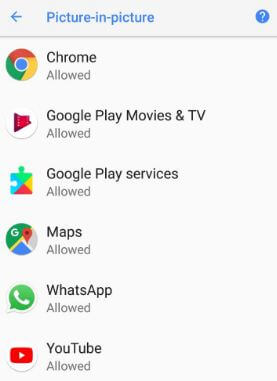This is a detailed screenshot of a mobile device's settings interface. The header features a gray background with a blue left-pointing arrow on the left side. Centrally positioned in the header is the label "Picture-in-Picture" displayed in blue text. On the right side, there is a dark blue circular icon featuring a white question mark. Below the header, a gray divider with a subtle shadow effect separates it from the main content area.

The main content area lists several apps along with their respective permissions. Starting from the top:

1. The Chrome icon appears on the left. To its right, "Chrome" is displayed in black text, with "Allowed" in gray text underneath.
2. Next, the Google Play Movies & TV app icon is shown. Beside it, "Google Play Movies & TV" is labeled in black, with "Allowed" in gray text underneath.
3. The following entry displays a puzzle piece icon for Google Play Services. To its right, "Google Play Services" is labeled in black, with "Allowed" beneath it in gray text.
4. A circular maps icon is next, featuring a green upper left segment with a white "G," a blue triangle at the bottom, a light gray left-pointing triangle, and a red map pin. To its right, "Maps" is labeled in black, with "Allowed" in gray text below.
5. The WhatsApp icon is shown, with "WhatsApp" to the right in black text and "Allowed" beneath it in gray.
6. Finally, the YouTube icon is displayed within a circular white icon featuring a rounded red rectangle with a white play button in the middle. To its right, "YouTube" is labeled in black text, with "Allowed" below in gray.

This screenshot succinctly displays various apps along with their Picture-in-Picture permission statuses.